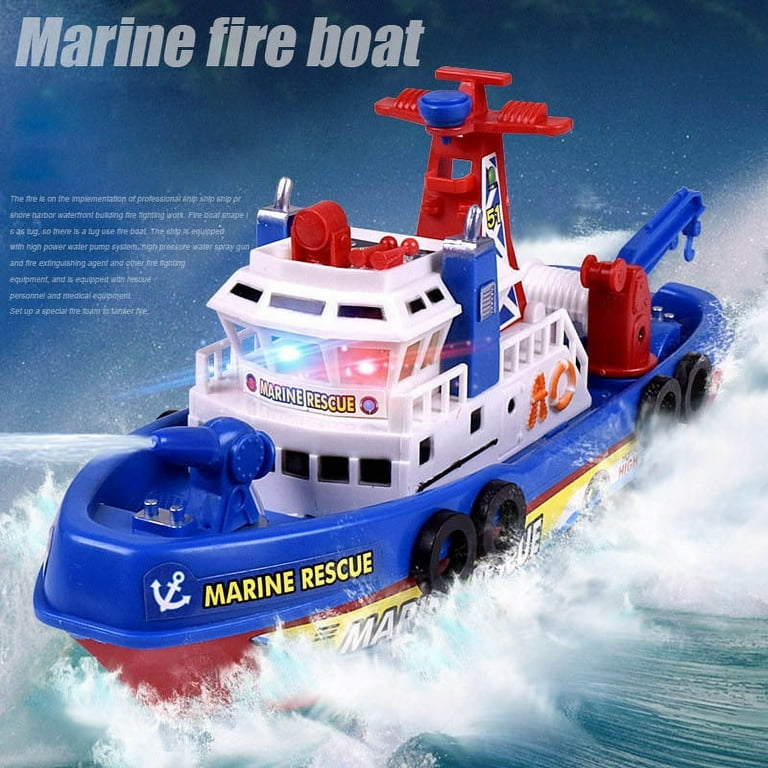This detailed photograph depicts a colorful plastic toy boat designed to resemble a marine rescue vessel, prominently featuring the label "Marine Fireboat" in the upper left corner. The image appears to be part of an advertisement, with the boat situated in a mock ocean scene with digitally added crashing waves. The predominantly blue deck houses a functional water cannon at the front, intended for firefighting scenarios. The boat's hull is vibrant red, mimicking the design of real-life rescue crafts. A white cabin, where the captain would be, features red and blue police lights, a red searchlight, and horns on the top. The boat is further equipped with a red and blue crane at the rear, used for hauling operations. Along the sides, there are black tires acting as bumpers, simulating docking scenarios. The entire setup of the toy is enhanced with a stormy sky background, adding drama and authenticity to the scene, making it an engaging representation for children. Although some descriptive text along the top side is too small to read, the deck also contains the label "Marine Rescue" in yellow, reinforcing the boat's purpose as a rescue vessel.